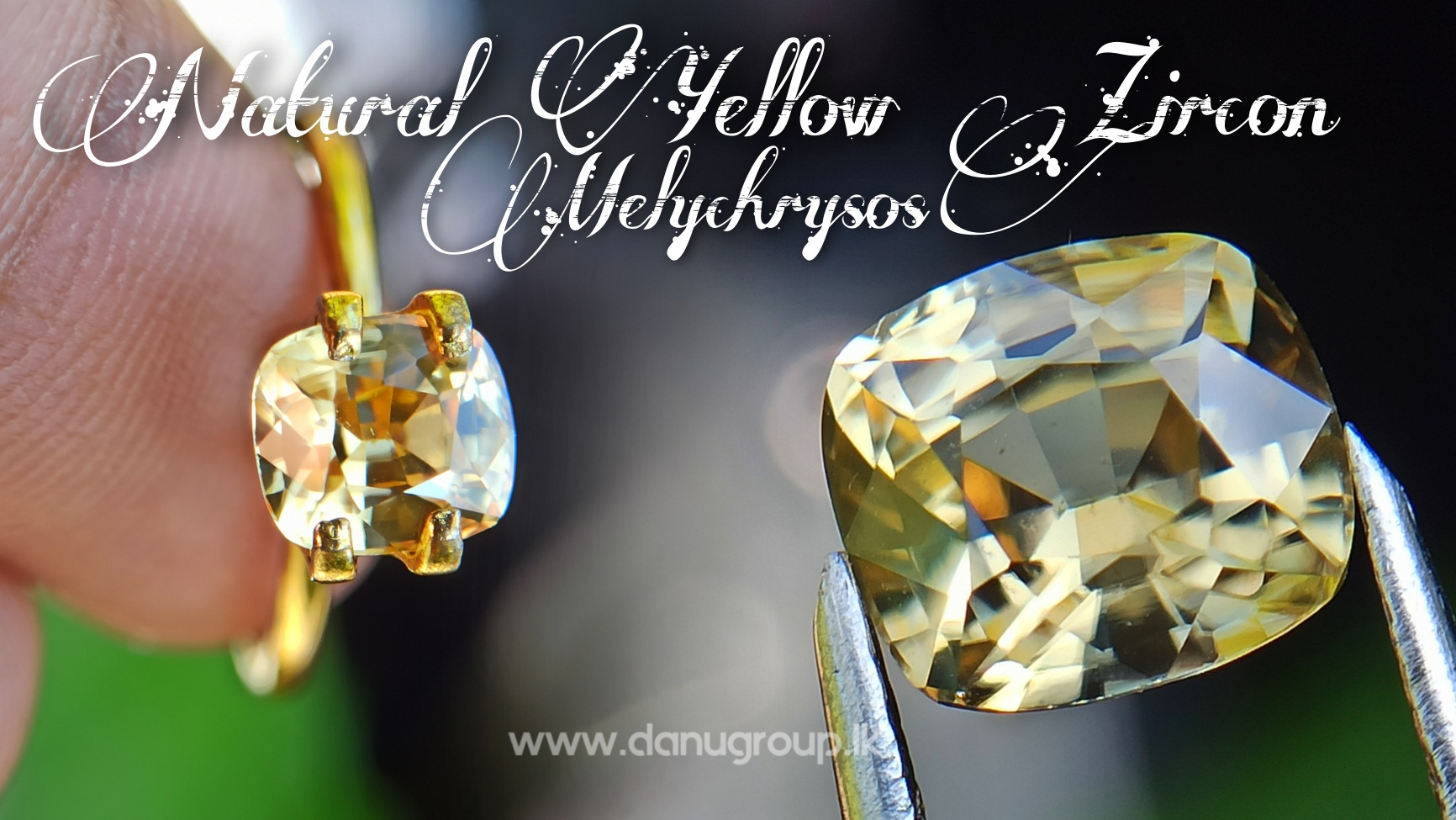This product image showcases two beautifully cut yellow zircon gemstones, emphasized by reflections of surrounding light that create black, orange, and gray highlights. The primary focus is on the right side, where a highly detailed, zoomed-in view of the gemstone reveals its numerous facets, held delicately by a pair of tweezers. Adjacent to this close-up, on the left, the same gemstone is set in a golden ring, being displayed by a finger. The image features a white cursive caption at the top that reads "Natural Yellow Zircon Melechrysos," while a transparent watermark at the bottom indicates the source as "www.danugroup.lk". The ring's golden band and the close-up of the intricate cuts on the zircon emphasize the high-quality craftsmanship of the piece, making it a stunning visual advertisement.